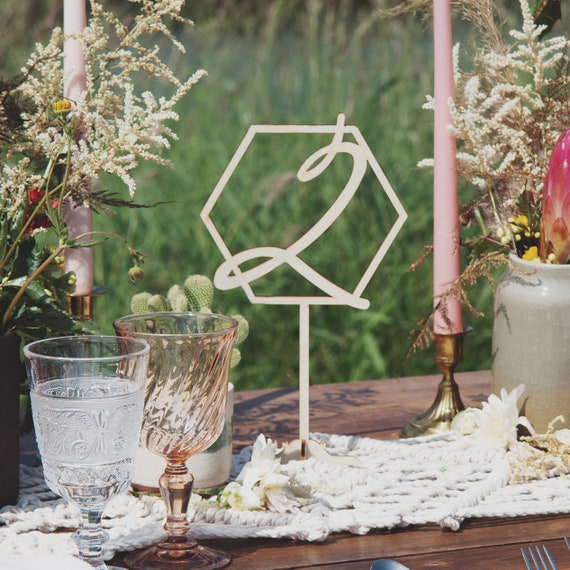In this close-up image taken outdoors on a picnic table, we see the detailed setting of a charming arrangement. The table itself is made of dark brown wood, with four horizontal planks. In the blurred background, lush green grass and various plants can be observed, suggesting a natural, serene environment.

On either side of the table, there are tall, pink candles held in elegant brass holders, with two floral arrangements—one of which is in a gray ceramic jug on the right side. These arrangements predominantly feature green and white flowers, with some red accents. The centerpiece on the table is a metal item with an octagonal shape, holding down a delicate white lace tablecloth. It has a scripted metal '2' affixed to it, hinting that this might be the second table setting for an event.

In the front left corner of the table, there are two wine glasses. One glass is clear with an opaque design and appears empty, while the other has a subtle peach hue. Tucked into the very corners of the table, a spoon and fork can be seen peeking out. This enchanting setting creates an inviting, intimate atmosphere perfect for a delightful outdoor meal.